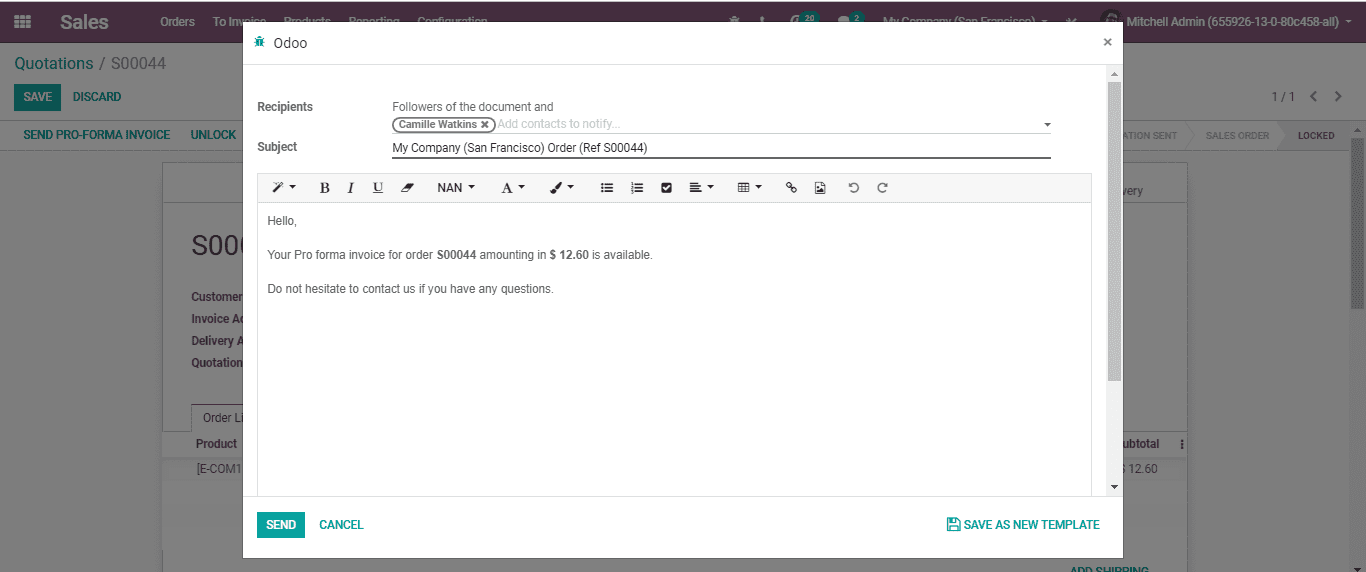This image shows a user profile belonging to Mitchell, who is affiliated with a sales department of a company based in San Francisco. The top of the profile screen partially displays navigational options from a sales management software, identified as an Odoo program. The visible options on the screen include "Sales," "Orders to Invoice," "Products," "Reporting," and "Configurations." 

Mitchell’s profile is labeled "Mitchell Administration" and is associated with the following numerical identifier: "655926-13-0-80-C458-ALL," with all text in lowercase. In the process shown, Mitchell is preparing to send an email message to a recipient named Camille Watkins. The email is directed to document followers and concerns a pro forma invoice related to order reference number S00044 from "My Company, San Francisco." 

The email message reads: "Hello, your pro forma invoice for order S00044 amounting to $12.60 is available. Don’t hesitate to contact us if you have any questions." 

The interface presents three options for the user: "Send," which is highlighted, "Cancel," and "Save as a new template."